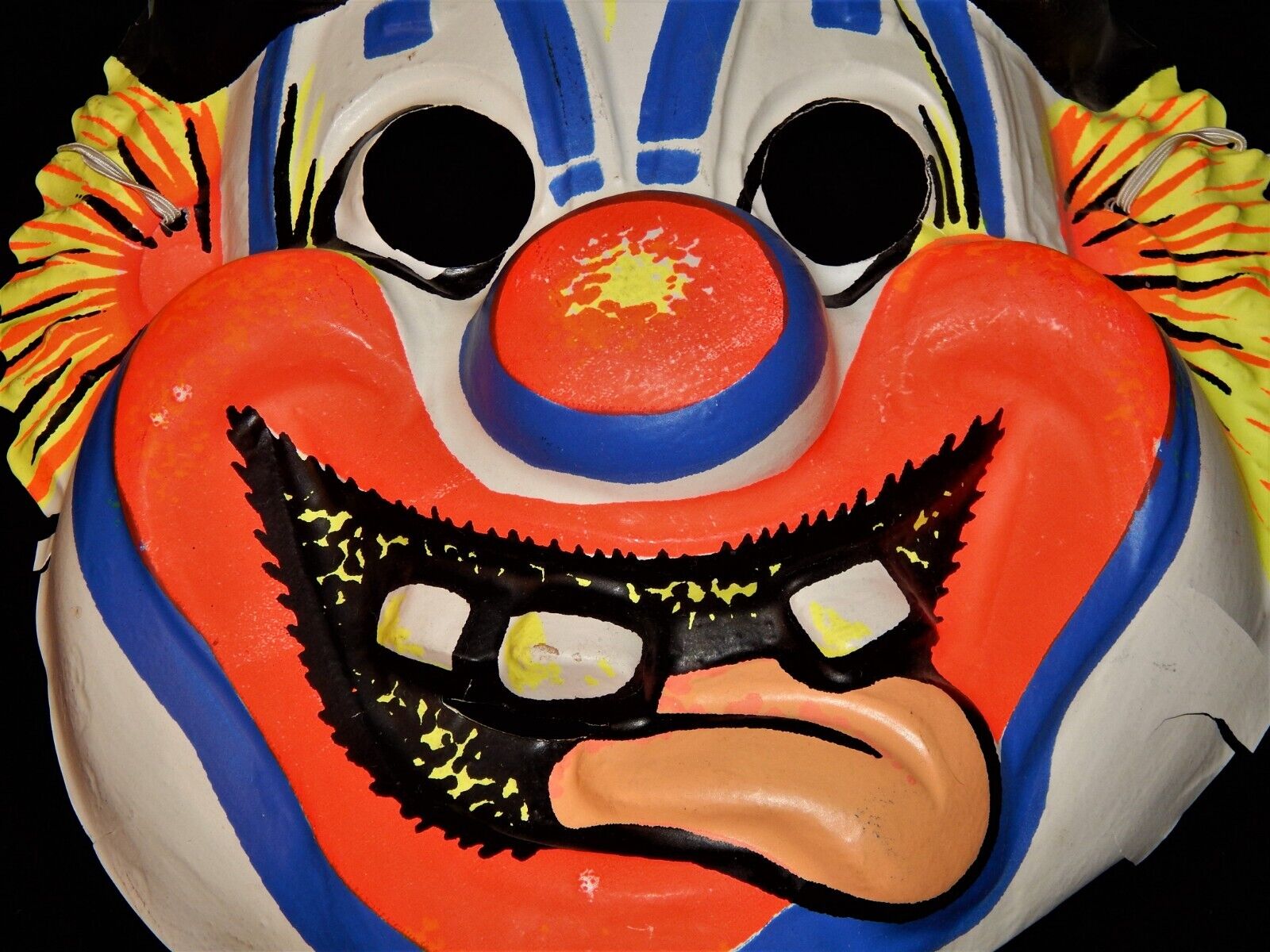This close-up photograph captures an aged, thin plastic Halloween clown mask, which dominates almost the entire frame, with only a small bit of black background visible in the corners. Central to the mask is a red nose with yellow specks in the middle, encircled by a broad cobalt blue border. Above the red nose are black eye holes framed by prominent M-shaped blue eyebrows. The mask is characterized by its vivid, frayed tufts of orange and yellow hair on the sides, resembling the fluffy feathers of a baby bird, and an attached strap visible at the back of the head.

The clown's exaggerated mouth, outlined in a mix of orangish-red and blue with a white border underneath, reveals a black interior and a missing front tooth among a set of three yellow-speckled teeth. A peach-colored, protruding tongue adds to the grotesque appearance. The entire mask shows signs of wear, with cracked and deteriorating edges, contributing to its eerie, vintage look from the 1970s. Despite its intended goofiness, the result is somewhat unsettling.